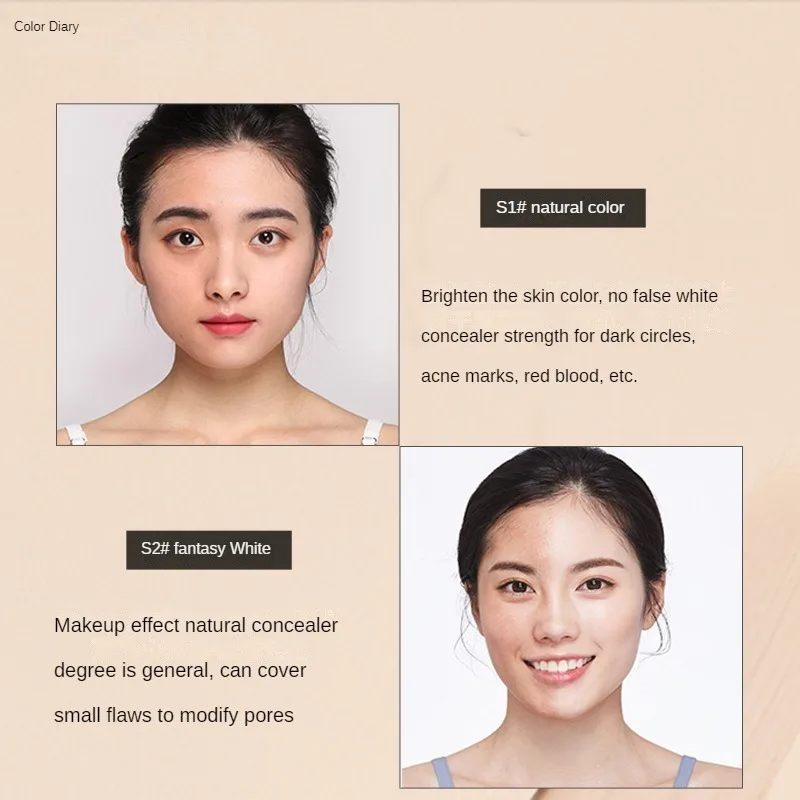The poster for a makeup product features a cream-colored background with the title "Color Diary" in small black letters in the top left corner. It is divided into two main sections. The top section features a photograph of a young woman of Asian descent with full reddish lips, dark hair, and dark eyes, looking pensively straight ahead. The text to the right of her reads "S1 Natural Color" inside a dark border in white letters, followed by descriptions in black letters that say, "Brighten the skin color. No false white concealer. Strength for dark circles, acne marks, red blood, etc."

Below this, to the right, there's another photograph of what appears to be the same woman, now smiling with paler skin, possibly due to makeup application. Next to this photograph, in black letters on the left, it reads "S2 Fantasy White" with additional text below stating, "Makeup effect: natural concealer degree is general. Can cover small flaws to modify pores." This suggests a before-and-after comparison, highlighting the effects of using the "Fantasy White" makeup product compared to the "Natural Color" option.